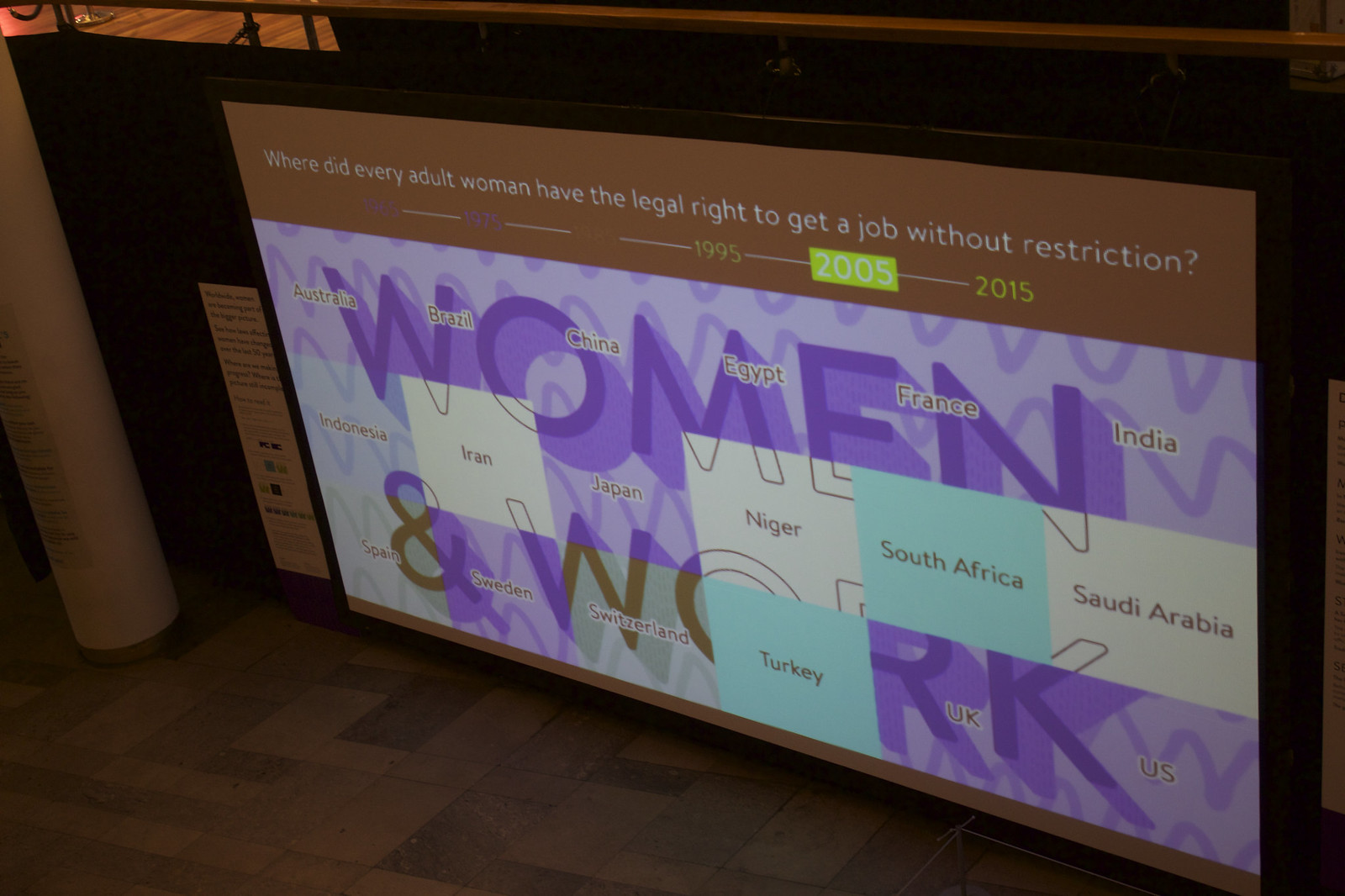This color photograph, taken indoors at a conference, captures an electronic display featuring a detailed discussion about women's legal rights in the workforce over the years. The lower portion of the image reveals a wooden floor while the upper section, about 15%, is darker and prominently displays a question in white text: "Where did every adult woman have the legal right to get a job without restriction?" Below this question, key years are listed: 1995, 2005, and 2015 against a purplish matte background with the phrase "Women and Work" written in large letters. The year 2005 is highlighted with a green background, indicating a significant point in the discussion. 

Displayed on this screen are the names of numerous countries, emphasizing their varied statuses regarding women's rights to employment. Countries include Australia, Brazil, China, Egypt, France, India, Indonesia, Iran, Japan, Niger, Saudi Arabia, South Africa, Spain, Sweden, Switzerland, Turkey, the UK, and the US. Specific countries are distinguished with unique colored boxes: South Africa and Turkey in light blue, Iran, Niger, and Saudi Arabia in white, Indonesia in light purple, and Spain and Switzerland in green, with others in the background of purple. The comprehensive list and color-coding provide a visual representation of global participation and progress in women's employment rights over the specified years.